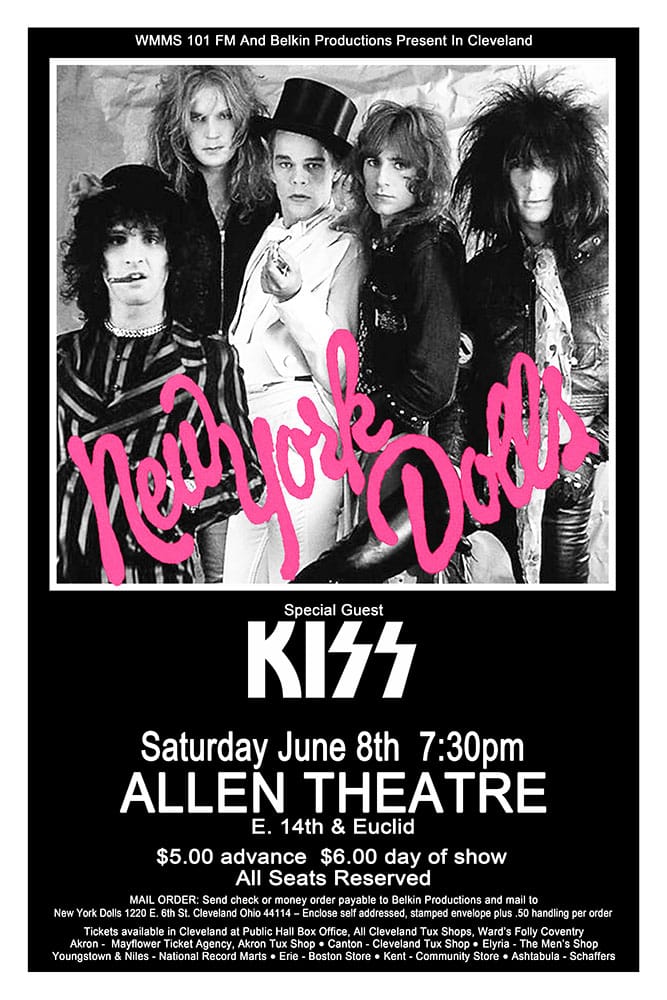The poster features a black-and-white theme with a striking hot pink cursive logo for the New York Dolls. It advertises a concert held on Saturday, June 8th at 7:30 p.m. at the Allen Theatre, located at East 14th and Euclid in Cleveland. The event is sponsored by WMMS 101 FM and Belkin Productions. The New York Dolls, a band likened to punk rock renegades with an appearance reminiscent of the late 70s scene, are prominently displayed in a photo dressed in flamboyant and over-the-top costumes, including a member wearing a top hat. The text details that tickets are $5 in advance and $6 on the day of the show, with all seats reserved. Additionally, the poster announces their special guest, the renowned rock band KISS, whose iconic logo is presented beneath the Dolls' image.